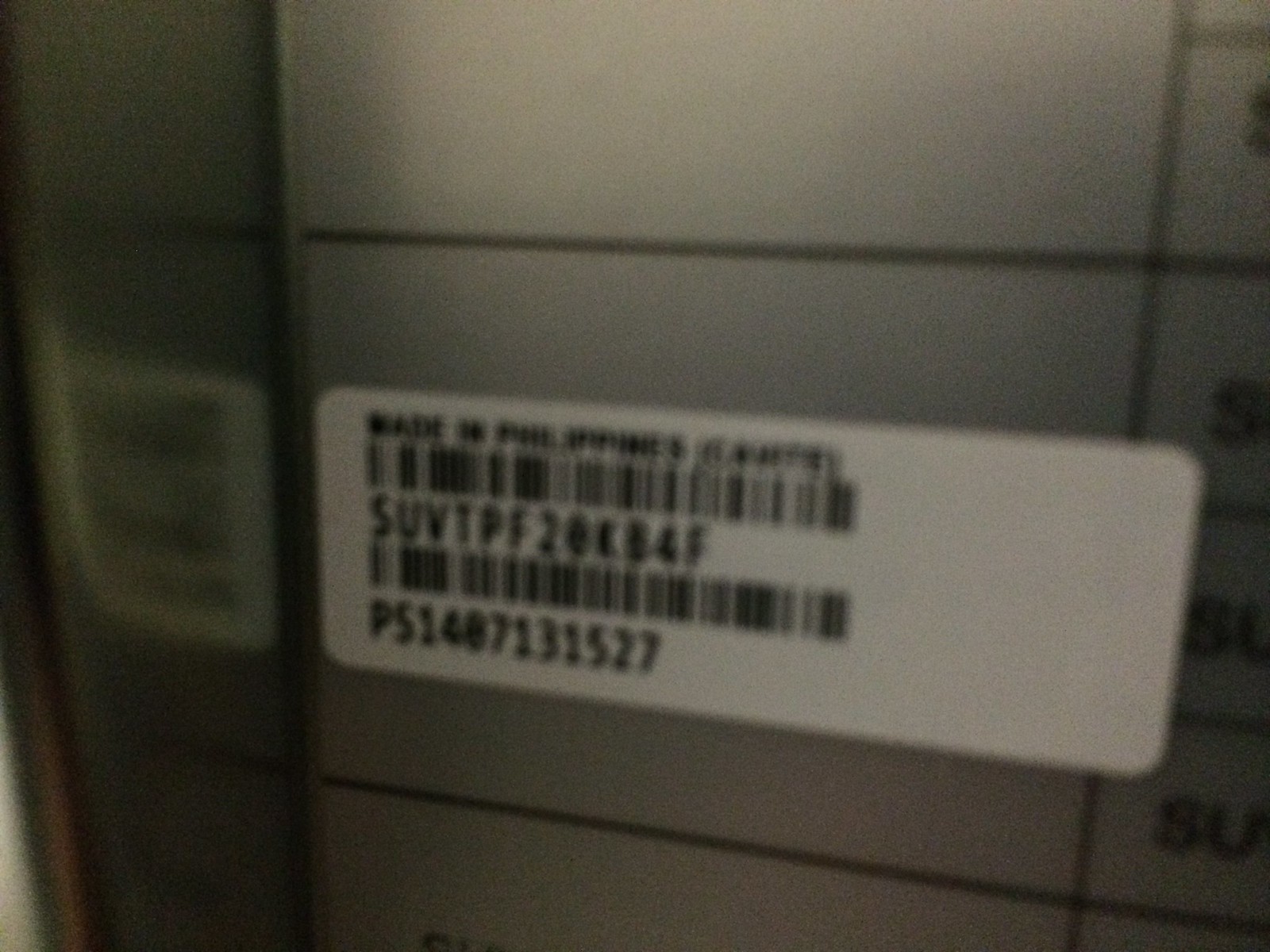This close-up photograph showcases a sticker affixed to a clear surface, prominently displaying two barcodes with corresponding numerical sequences beneath each. The sticker features the text "Made in Philippines" at the top. A third, vertical barcode appears on the left side of the image, although it is notably blurred and out of focus. The backdrop consists of a white surface segmented into rectangles, containing partially visible, cut-off text along the right edge of the photo. The rectangular lines seem slightly angled towards the left, suggesting the photo was taken at an angle. The overall image is tinged with gray and exhibits a certain fuzziness, indicating a lack of high resolution. The capture appears to serve a practical purpose, likely intended to share the barcode details for identification or verification of a part.